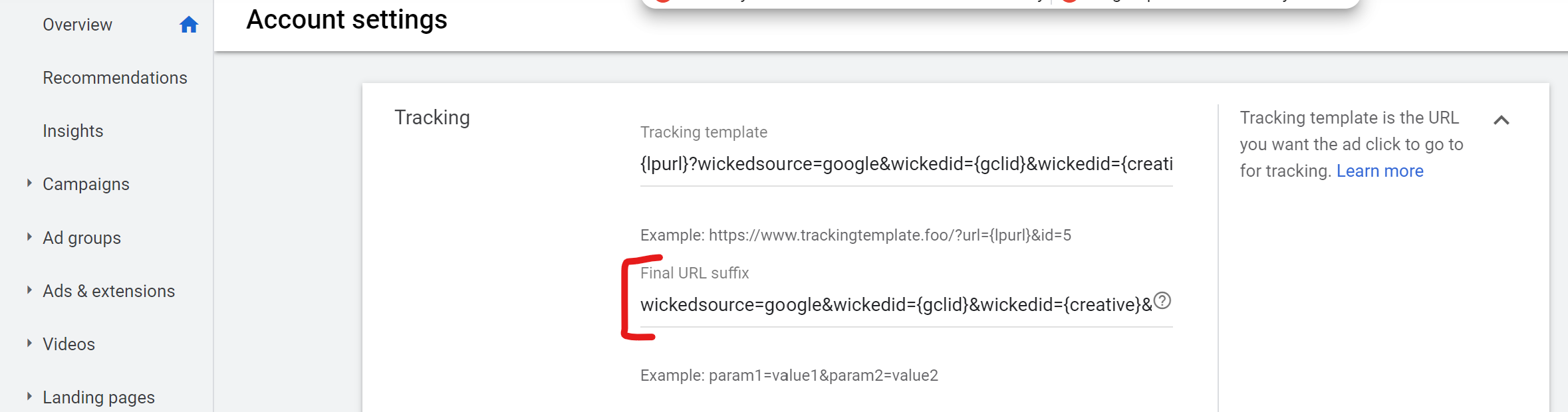This screenshot captures a section of a computer screen displaying a web interface with a distinct layout. On the left side, a gray sidebar lists several navigation options in a vertical manner: "Overview" (adorned with a home icon to its right), followed by "Recommendations," "Insights," "Campaigns," "Ad Groups," "Ads and Extensions," "Videos," and "Landing Pages."

Adjacent to the "Overview" label, the text "Account Settings" is visible towards the right. 

In the center of the white background area, the heading "Tracking" is located in the top-left corner. To its right, the term "Tracking Template" is displayed, followed by a brief description: "Tracking template is the URL you want the ad click to go to for tracking." 

A blue hyperlink labeled "Learn more" is shown further to the right.

Below this section, back on the left side, there is the word "Example," followed by a URL using the HTTPS protocol. Positioned beneath this, the label "Final URL Suffix" appears, with the content "wicked source equals Google Wicked, E-D-I-D" encased within red brackets. An example follows immediately below this text. The remaining part of the screen retains a white background, offering a clean visual focus on the detailed elements described.